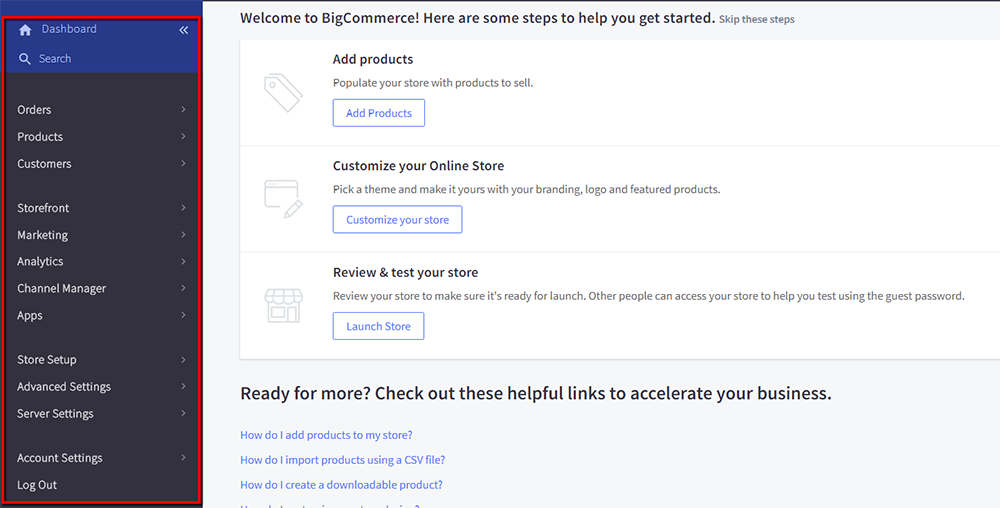In the image, there is a sidebar on the left side of the screen, segmented into distinctly colored sections. The top part of the sidebar features a dark blue background with a house icon labeled "Dashboard" and a magnifying glass icon representing "Search". Below this, the sidebar transitions to a black background, listing various categories in white text: "Orders", "Products", "Customers", "Storefront", "Marketing", "Analytics", "Channel Manager", "Apps", "Store Setup", "Advanced Settings", "Server Settings", "Account Settings", and "Logout". Each category is accompanied by a clickable greater-than symbol (>) to its right. The entire sidebar is outlined in a red box, indicating it has been edited or highlighted for emphasis.

On the right side of the image, there is a welcome message from BigCommerce, stating, "Welcome to BigCommerce! Here are the steps to help you get started." Following this introduction, users are given the option to "skip these steps." The first step is "Add Products: Populate your store with products to sell," accompanied by a blue button labeled "Add Products." The second step encourages users to "Customize your online store: Pick a theme and make it yours with your branding, logo, and featured products."